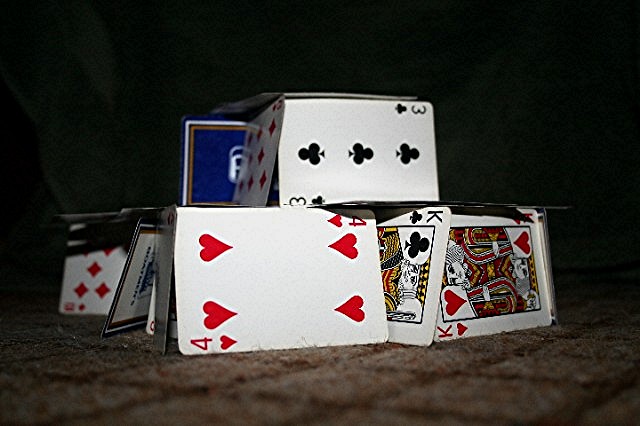The image features a dimly lit scene with a dark background, highlighting a carefully arranged stack of playing cards on a grayish-brown carpet or rug. The cards form a two-story structure, reminiscent of a small card tower. On the lower level of the arrangement, visible cards include the Four of Hearts, the King of Clubs, and the King of Hearts. The upper level of the structure showcases three cards from the Clubs suit and an unidentified Diamond card placed to the side, its value obscured. Despite the overall lack of lighting, the arrangement and details of the cards are clearly discernible.